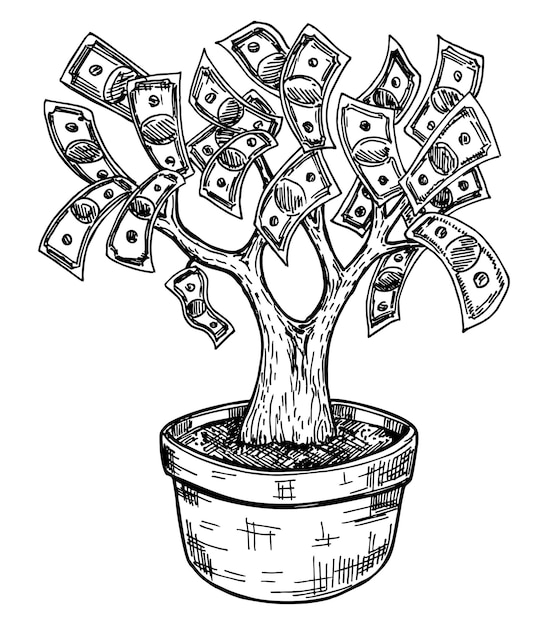This black and white pencil sketch depicts a "money tree" planted in a pot. The pot, drawn with detailed cross-hatching to indicate texture, sits on the ground filled with soil. The tree's trunk is robust and textured with detailed line work to suggest the roughness of its bark. It branches out into two main limbs that further subdivide into several smaller branches. Instead of leaves, the branches are adorned with paper money bills. While the bills lack detailed designs, their rectangular shape and faintly indicated central face suggest dollar bills. The overall drawing is simplistic yet detailed, with careful shading and line work to emphasize the different textures of the pot, bark, and bills.